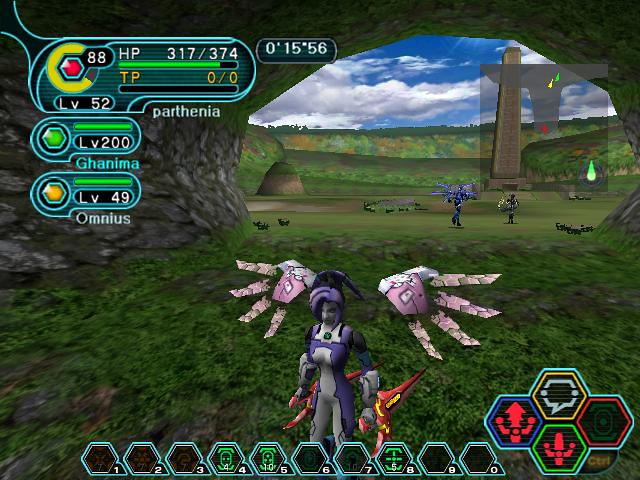In this video game scene, the screen displays various game stats such as score, levels, and lives in the upper left-hand corner. The main visual depicts a lush, green environment leading into a cave. At the cave's entrance, where the ground is covered in moss or grass, stands a character dressed in purple. Surrounding the cave opening are jagged rocks and stalactites, enhancing the natural, rugged appearance. Additional characters are visible approaching the cave, all set against a backdrop of a blue sky bustling with white clouds, adding depth and contrast to the vibrant scene.